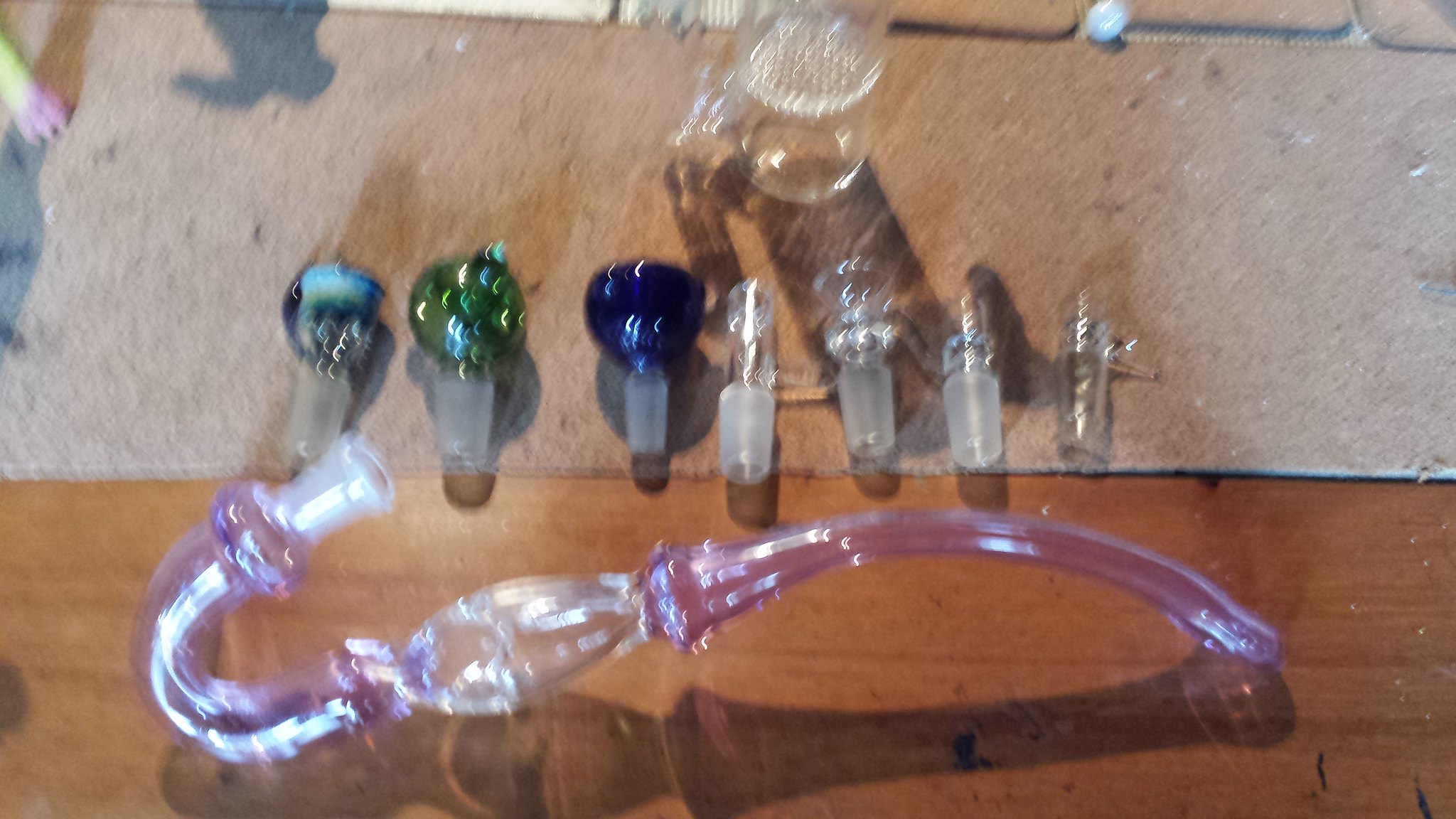A very out-of-focus, top-down photograph shows a collection of approximately nine blown glass pieces likely intended for use with bongs or pipes. Among the items are several bowl pieces with a non-shiny, tapered surface possibly designed for fitting or replacement purposes. The centerpiece appears to be a glass pipe with a curved, saxophone-like structure made of pink and clear glass. The photo captures these items placed on a floor where finished wood meets a dirty, carpeted area, accentuating the scattered dirt and casting shadows. Colors vary among the pieces, including blues, greens, and clear glass. The blurred image suggests the camera was possibly moved during the shot, further complicating visual clarity amidst poor reflections and peculiar shadows.